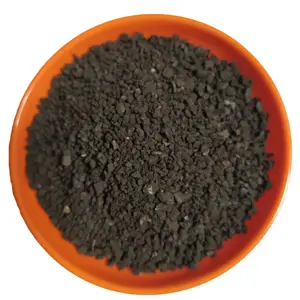The image depicts an orange ceramic dish with a gradient coloring, lighter on the top left and darker towards the bottom right, against a white background. The rim of the dish is a lighter shade compared to its vibrant interior. Inside the dish, occupying almost its entire 12-inch diameter, is a brown substance that might be soil, coffee powder, or possibly black granules or finely chopped pieces of chocolate. This substance is primarily brown in color, with white speckles interspersed throughout. The focus of the photograph is sharper at the center of this granular material, while the edges, especially on the left side, appear blurred, making the central area more detailed and prominent.